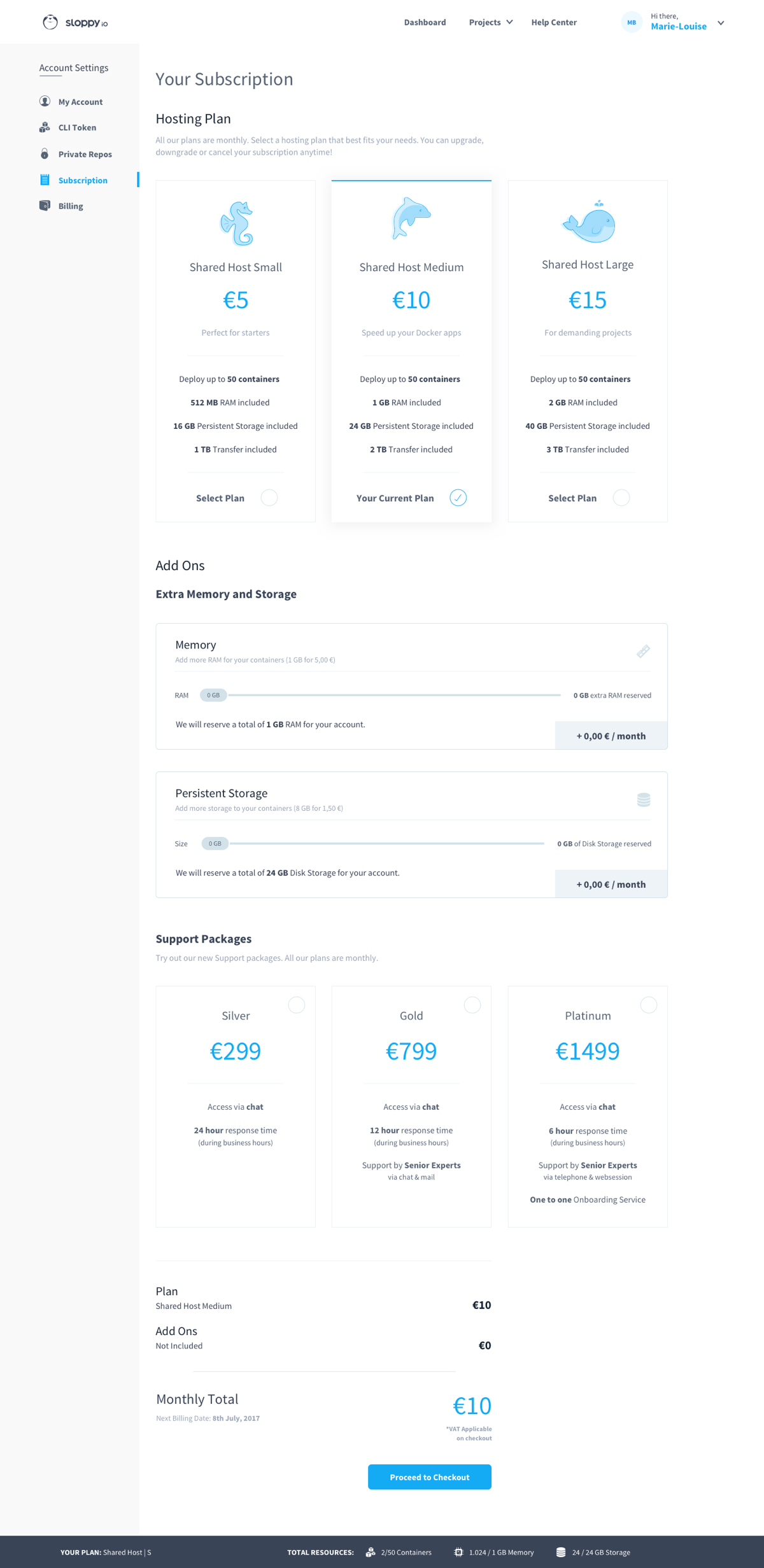The webpage displayed appears to belong to a website called "Slotty" or possibly "Sloppy," and showcases various hosting plans available for purchase. The layout is set against a predominantly white background with blue highlights, providing a clean and visually appealing design. 

At the forefront are three distinct hosting plans, central to the webpage:

1. **Shared Host Small**: Priced at €5, this plan includes a specific amount of storage and features. It is represented by a blue seahorse icon. Although the text is somewhat blurred, it indicates the plan's allocated space.

2. **Shared Host Medium**: This highlighted plan costs €10 and offers more storage and features than the small plan. Its icon is a blue dolphin. The detailed text is slightly zoomed out, but it suggests enhanced capabilities.

3. **Shared Host Large**: Available for €15, this plan provides the most resources among the three and is symbolized by a charming blue whale icon.

Beneath these plans, there are options for add-ons such as additional memory and storage, adjustable via a slider to customize the amount needed. 

Moreover, there are support packages outlined:

- **Silver Support**: Priced at €2.99
- **Gold Support**: Priced at €7.99
- **Platinum Support**: Priced at €14.99

Each support package offers varying levels of service, though the specific details are not fully visible.

The current selection on the page is the "Shared Host Medium" plan at €10, with no additional add-ons chosen. At the bottom, the total monthly cost is displayed, accompanied by a button to proceed to checkout.

At the top of the page, there are account management options indicating that the user is logged in, with links to view account settings and subscriptions.